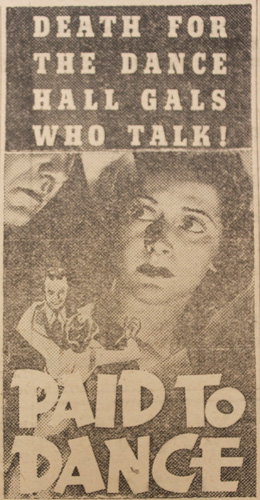The image is a vintage advertisement likely hailing from the 1930s or 1940s, possibly promoting an old exploitation thriller film. The ad has a black and white color scheme, printed on faded beige paper with a dot matrix printing style, suggesting it might have originated from a newspaper. The top of the ad features a prominent black text box with bold white serif text proclaiming, "DEATH FOR THE DANCE HALL GALS WHO TALK." Below this text is a detailed, dramatically lit painting of a young woman gazing nervously over her shoulder, with noticeable shadows on her face. Behind her, a stern-faced man looms closely. Highlighting the period's style, the woman has a 1950s hairdo and dark lipstick. The bottom section of the ad showcases an illustration of a man and woman dancing, which serves as a backdrop to the film's title, "PAID TO DANCE," displayed in a bold, funky font. The overall faded look and brownish tones of the ad contribute to its vintage and somewhat lurid appeal.